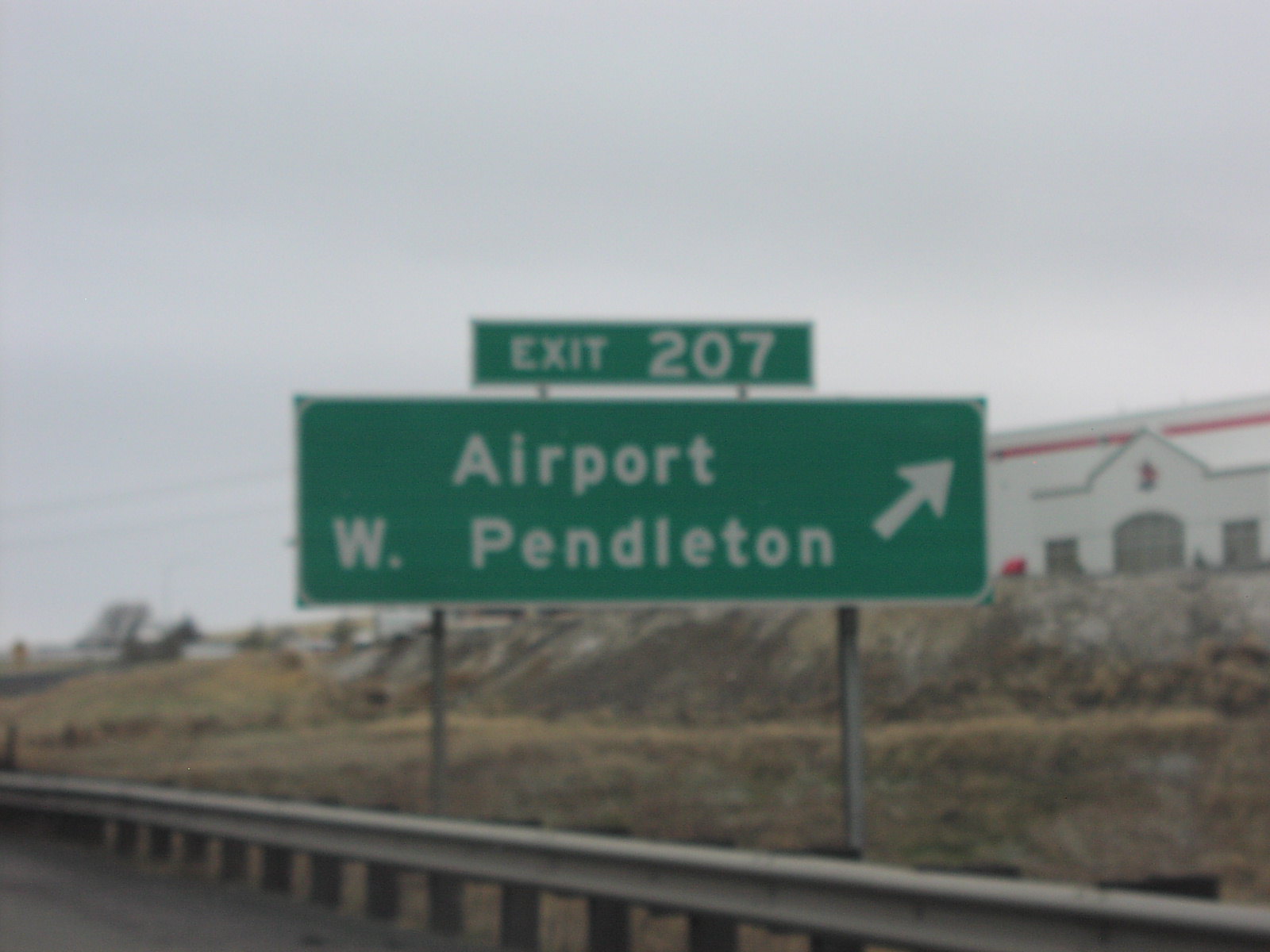This outdoor photograph features a centered pair of street signs, captured with noticeable blurriness and low quality. At the top of the image, a small, rectangular sign with a green background reads "EXIT 207" in white text. Directly below, a larger rectangular sign, also with a green background, displays the words "AIRPORT" followed by "W. PENDLETON" underneath, alongside an upward-pointing arrow. The signs are supported by a pair of poles positioned on either side, providing structural support. Despite the poor image clarity, the signs remain legible and provide directional guidance for travelers.